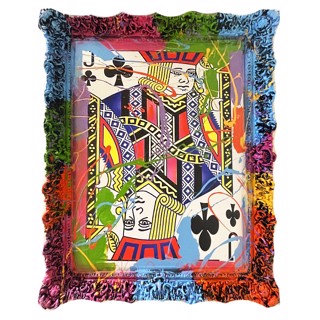This vibrant vertical image features the Jack of Clubs playing card enveloped in a vividly colorful frame. The card's iconic elements, such as the black "J" and club symbol, stand out against a white background. The Jack himself is adorned with a red crown accented with blue, has yellow hair, and a white face. His attire is a rich medley of red, blue, black, yellow, and purple. The frame alternates its bright colors in a striking pattern, incorporating blue, pink, green, yellow, purple, and red, with loops and circles blending into each other. These vivid hues spill over and overlap the boundaries of the card, creating a painted and slightly chaotic look. The design appears intentional, adding an artistic, almost splashed-paint quality to the entire piece.